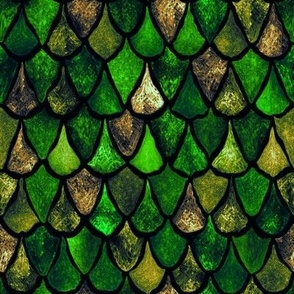The image is a detailed, close-up pattern resembling a mosaic of overlapping, triangle-shaped tiles, reminiscent of both fish scales and roof shingles. These tiles are primarily in varying shades of green, from dark, emerald tones to lighter, almost glowing hues, with some interspersed darker, silvery, and brownish elements. Each triangular tile is outlined in black, and together they create a harmonious yet intricate design. The pattern alternates like an array of upside-down and upright ice cream cone shapes, evoking the aesthetic of a stained glass window. One tile towards the top is notably lighter, almost white, suggesting a translucent effect as if light is shining through it. The entire image is free of text or other objects, emphasizing the detailed and luminous quality of the green tiles.